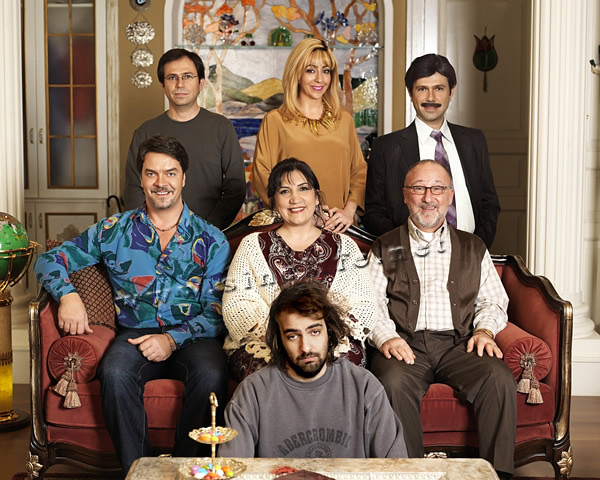The photograph captures a detailed family portrait set in a modern yet ornate living room. The group is arranged in three rows. At the front, a bearded man with long hair, looking quite unhappy, sits on the floor wearing a gray Abercrombie sweater. Behind him, seated on an orange-red sofa, are three people: a joyful man on the left, a woman in the center, and an older gentleman on the right. The third row features three more standing individuals: another man on the left, a woman in the middle, and an additional man on the right. Everyone, except the frontmost gentleman, is smiling. The room’s focal point includes a colorful painting hanging on the wall behind them.